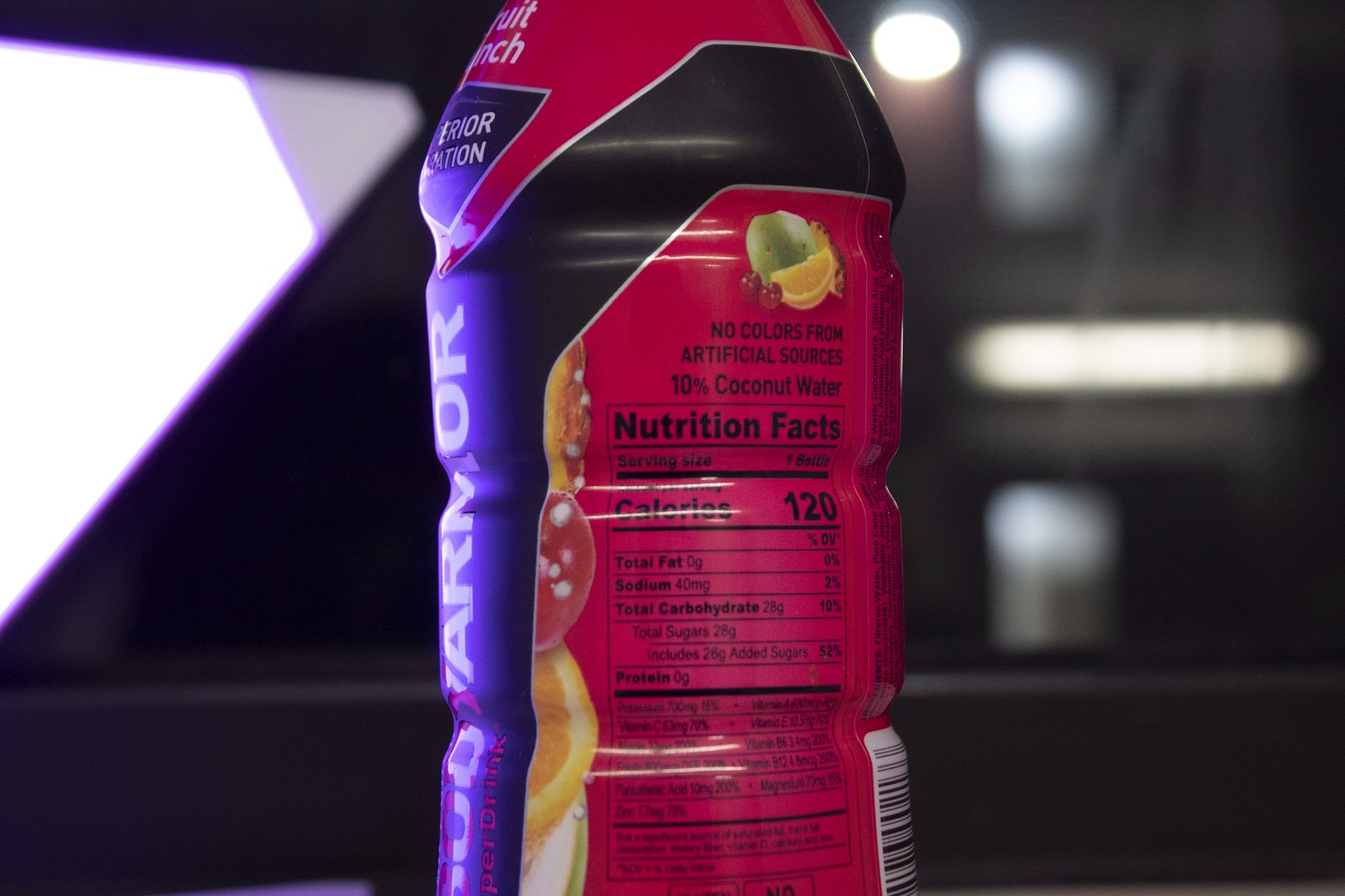This photograph captures the back of a uniquely textured beverage bottle. The bottle's surface features a series of notches and ridges, creating an interesting, contoured appearance. The label, which wraps around the bottle, includes a distinct red section showcasing nutritional information. At the top of this red section, there are vibrant images of fruits, including a lime, an orange slice, and cherries, likely indicating the flavors or ingredients of the drink. Prominent text on the label highlights that the product contains no colors from artificial sources and includes 10% coconut water. The nutrition facts box reveals that the drink contains 120 calories. On the left edge of the label, partially visible text displays the word "Armor," hinting at the brand or type of the beverage.